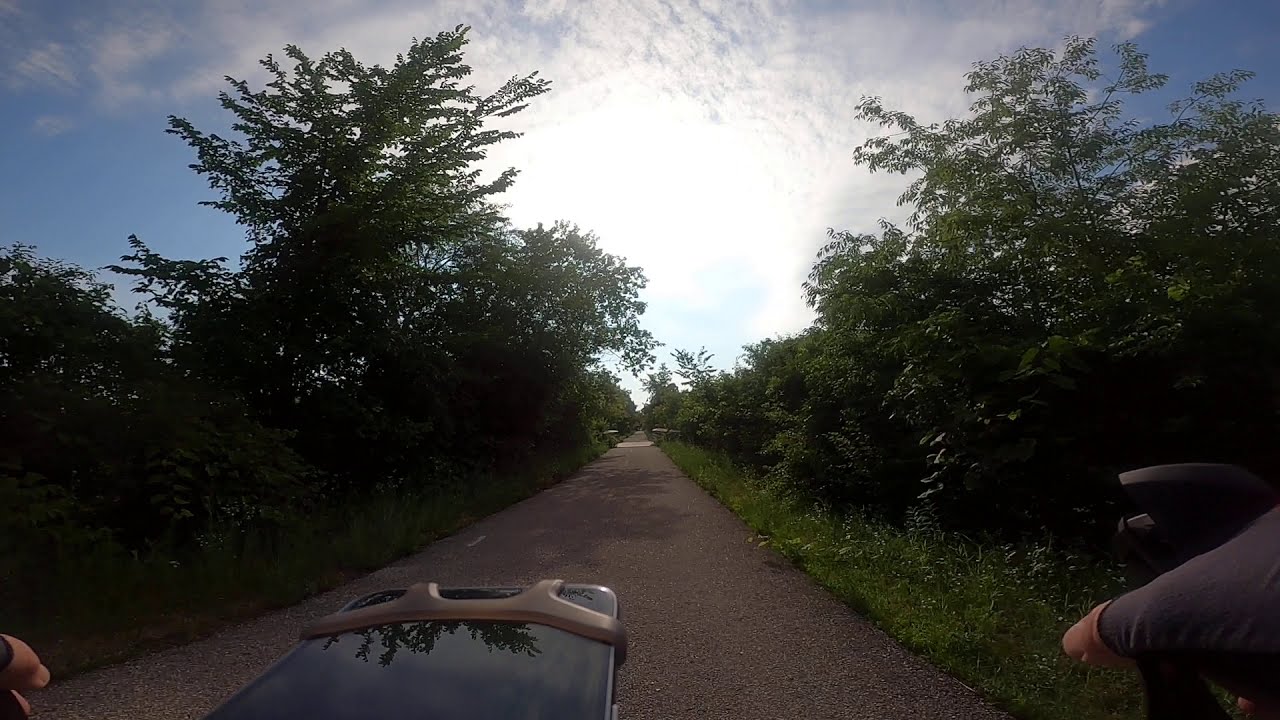The image captures a first-person perspective from someone riding a mountain bike on a well-maintained, paved trail. Prominently, a phone is mounted in the center of the handlebars, its dark screen reflecting the bright blue sky dotted with white, diffused clouds overhead. The rider's hands are barely visible on either side, gripping the handlebar. Surrounding the path, which stretches straight ahead, is lush green grass and overgrown greenery flanked by tall trees. The day appears semi-cloudy yet brightly lit, enhancing the natural outdoor setting. The scene reflects hues of brown, black, green, tan, blue, gray, and white, depicting a tranquil moment in nature.